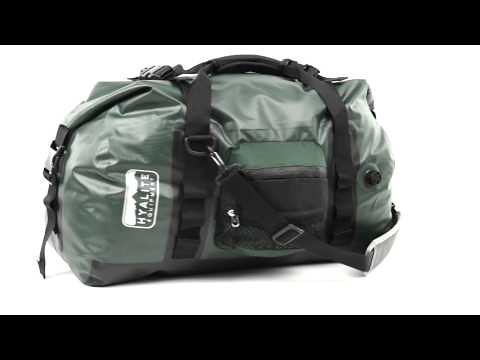This is a detailed photograph of a tactical duffel bag, likely used for heavy-duty travel or survival purposes. The duffel bag is crafted from a robust dark green synthetic material, possibly canvas or vinyl, known for its durability and resistance to scratches and tears. It features multiple carrying options, including a shoulder strap and black suitcase-style straps for versatility. In the front, there is a square pouch for additional storage, alongside other compartmental pockets designed to hold smaller items securely. The bag prominently displays the logo of "HiLit Equipment" in white, though some of the text is slightly blurry. The background of the image is plain white, and it has black borders on the top and bottom, suggesting this could be a screenshot from a video in widescreen aspect ratio. This duffel bag does not cater to luxury but is tailored for rugged use, potentially including features like a specialized pocket for carrying water, making it ideal for camping or survival scenarios.